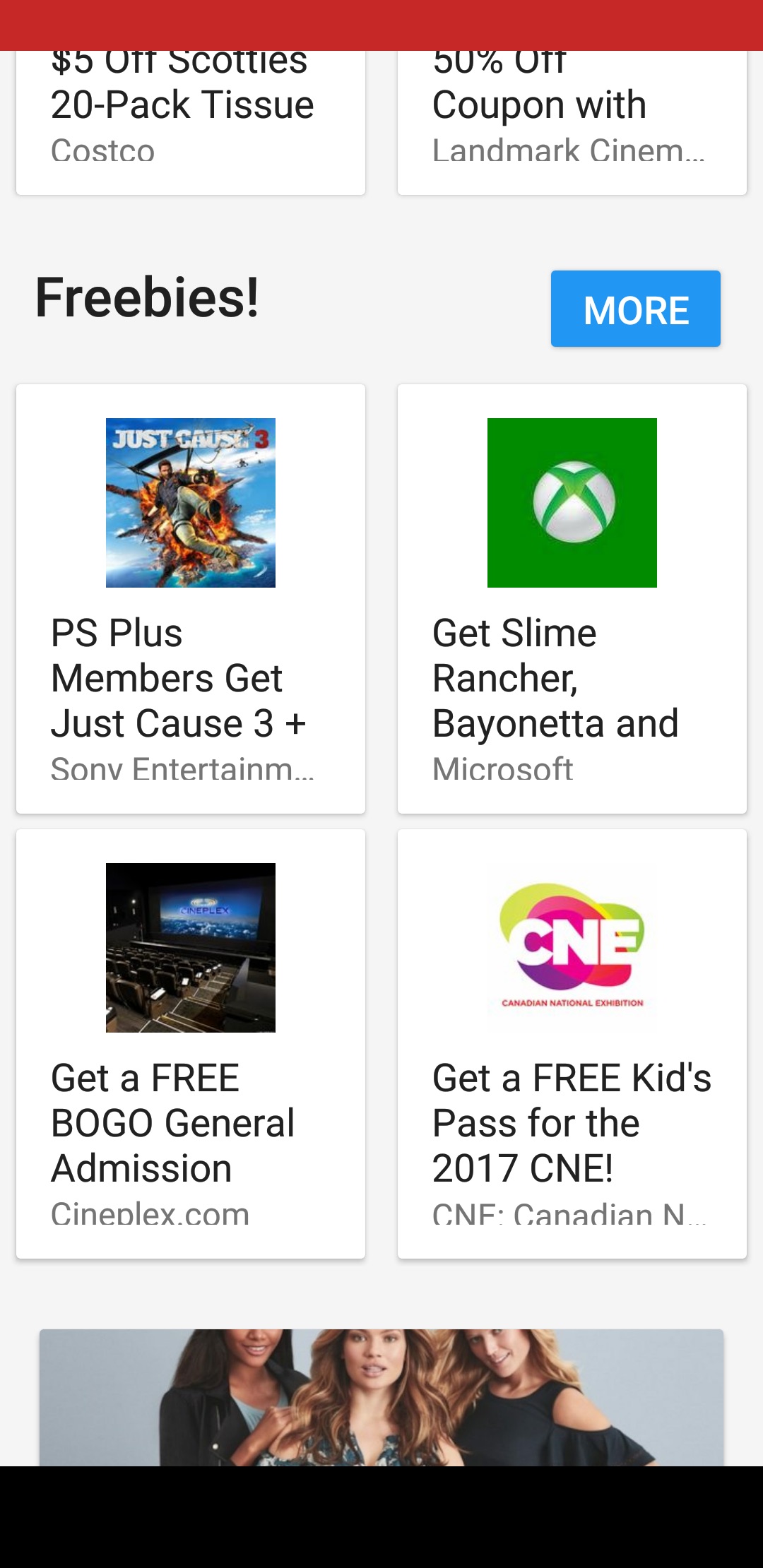The screenshot captures the display of a phone screen in mid-scroll, revealing a variety of promotional offers and discounts. Visible at the top is a prominent red bar, below which several coupon deals are shown. The first highlighted offer provides "$5 off Scotty's 20-pack tissue" at Costco, followed by a substantial "50% off at Landmark Cinemas." Additionally, a "Freebies" section is evident, with clickable options for more details.

In the "Freebies" section, the initial offer is for PS Plus members, who can obtain the game "Just Cause 3" at no extra cost. Other enticing offers include "Slime Rancher" and "Bayonetta" games, identified with an Xbox 360 symbol, suggesting they are available for Microsoft users. Furthermore, there's a "Buy one get one free" general admission offer from cineplex.com and a free kids pass for the 2017 Canadian National Exhibition (CNE).

Part of the screen also shows an image of three women with a black bar below them, though the context or purpose of this image is not clear from the visible portion of the screen.